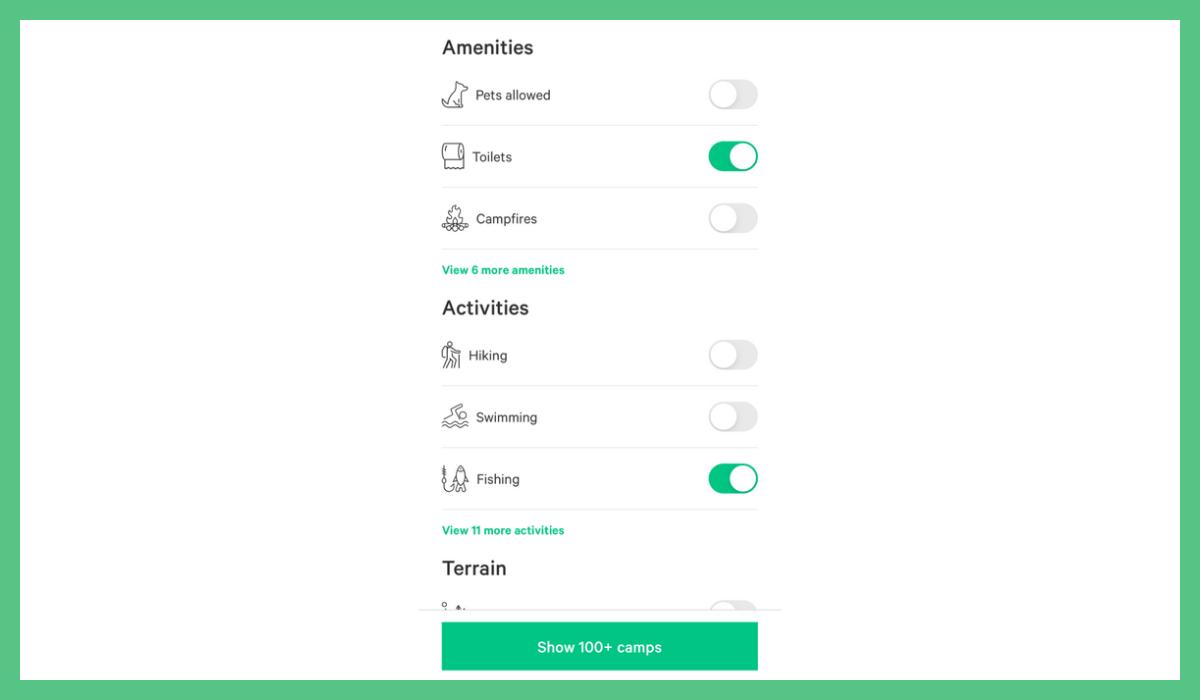This is a detailed screenshot of a website designed to help users find camps based on selected parameters. The main content is framed within a white rectangle bordered by a green outline. 

At the bottom of the image, there is a prominent green button with white text that reads, "Show 100+ camps." 

At the top of the image, centered text and elements indicate the primary focus areas of the filtering system. The first clearly defined section labeled "Amenities" in black text features options such as "Pets Allowed," "Toilets," and "Campfires." Each amenity is accompanied by toggle switches to filter results based on user preference. The "Toilets" option is currently activated, as indicated by its green switch, while the other options remain gray. Below these options, a green hyperlink reading "View 8 more amenities" invites users to explore additional amenities.

The next section is titled "Activities" and includes options such as "Hiking," "Swimming," and "Fishing," again with a green link beneath that states, "View 11 more activities."

The final visible section is labeled "Terrain," but the full details of this section are not shown, suggesting that more options continue further down the page, beyond the visible portion of the screenshot.

Overall, the layout appears user-friendly, organized into sections with concise labels and interactive elements for an efficient camp-finding experience.